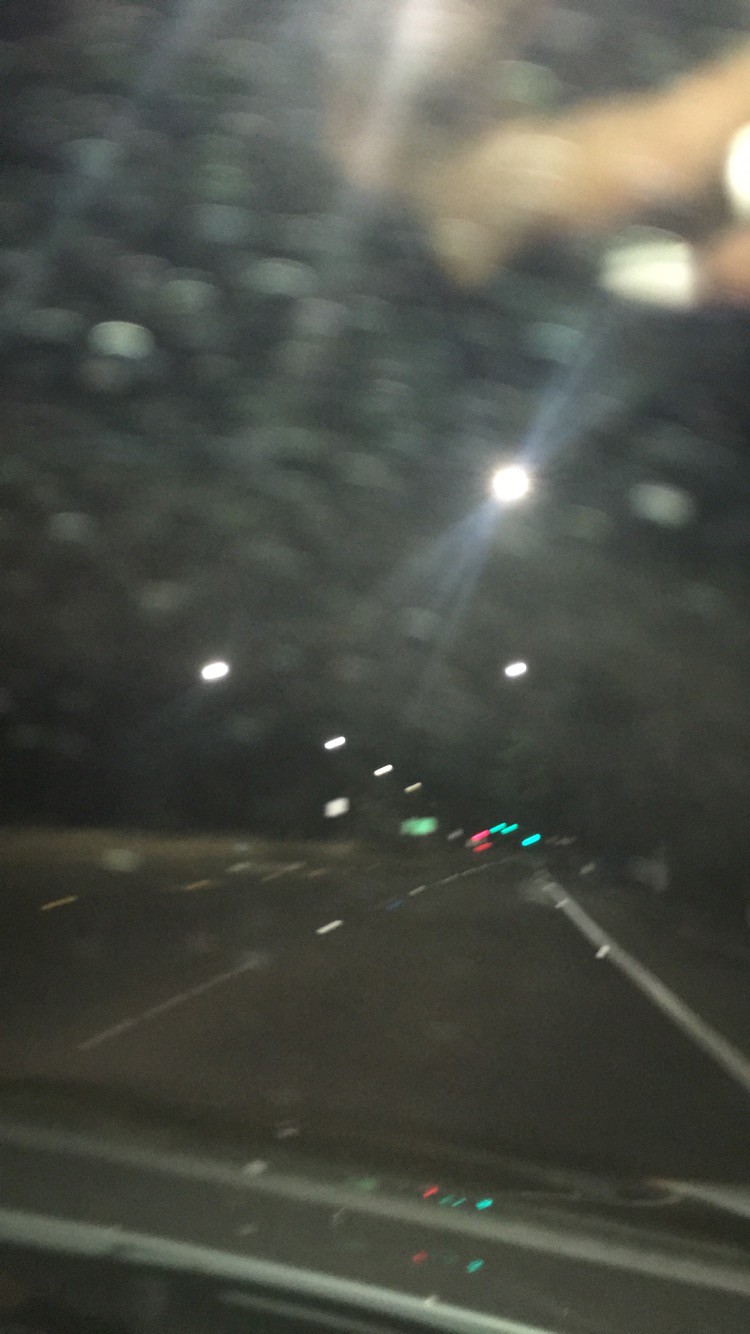Through the rain-streaked windshield of a car, an out-of-focus nighttime scene on a three-lane highway unfolds. The image is slightly blurry as raindrops scatter across the glass, with the car’s wipers resting idle. Despite the poor visibility, the distant highway is discernible, illuminated by overhead street lights and sidelined by traffic markers. The central stripes of the highway are visible through the rain, with a solid white line marking a reserved lane on the far right side. To the left, dashed lines demarcate the lanes. The car's dashboard is partially visible at the bottom of the frame, adding to the context of a stormy night drive along a wet and glistening roadway.